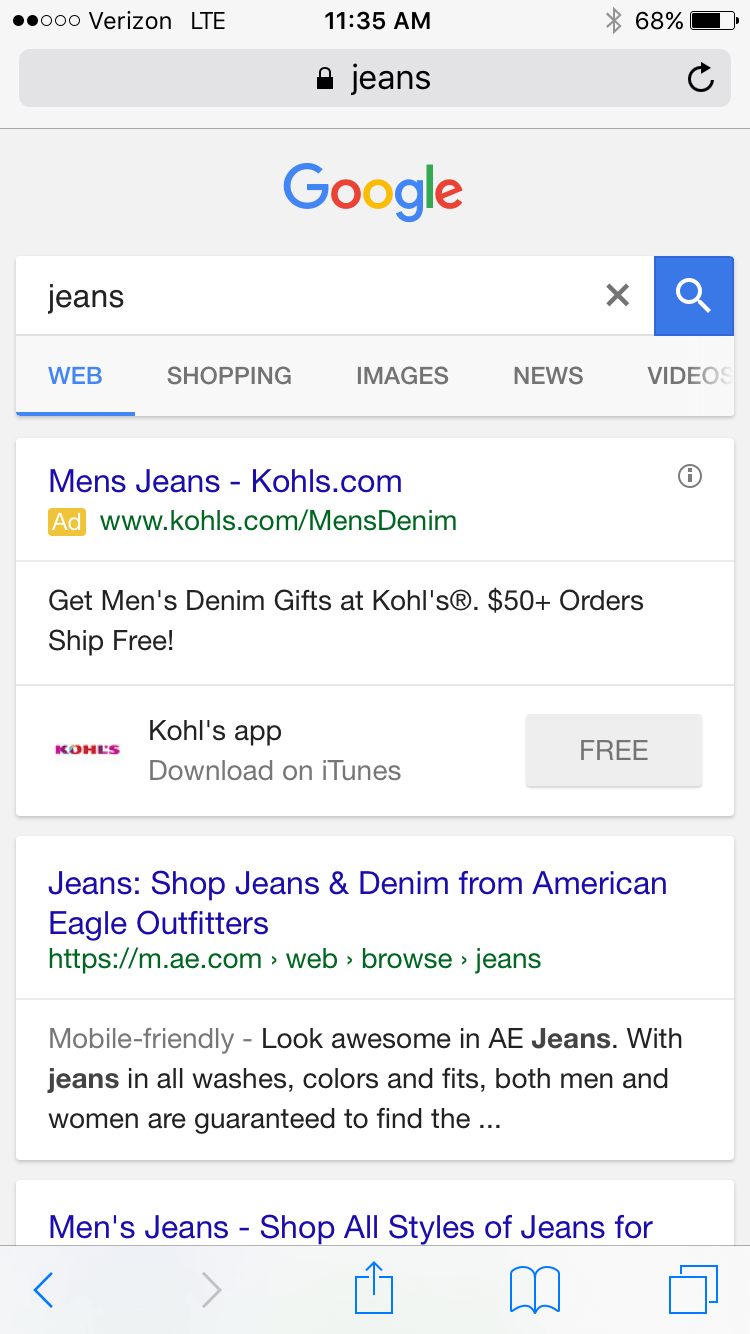This image showcases a cell phone screen displaying a Google search for "jeans." In the top left corner, the cellular network is identified as Verizon LTE. The time, 11:35 AM, is centered at the top, while the top right corner features the Bluetooth icon, the battery level at 68%, and a battery image.

Just below this, a Google search bar displays the word "jeans." Following the Google logo is another search box also containing the word "jeans," with the "Web" tab highlighted next to options for "Shopping," "Images," "News," and "Videos." The search results section lists three entries.

The first search result is from "mensjeanskoles.com," labeled as an ad. The brief description reads, "Get men's denim jeans at Kohl's. $50+ orders ship free." Accompanied by the Kohl’s logo, there is a prompt to download the Kohl's app on iTunes, including a button labeled "Free."

The second search result links to American Eagle Outfitters, with the description, "Shop jeans and denim from American Eagle Outfitters." It mentions that the site is mobile-friendly and encourages shoppers with, "Look awesome in AE jeans with jeans in all washes, colors, and fits. Both men and women are guaranteed to find the..."

The third search result, partially cut off by the bottom of the phone screen, begins with "mensjeans, shop all styles of jeans for." 

At the very bottom of the screen, navigation icons are displayed: a left-pointing arrow, a right-pointing arrow, a box with an upward-pointing arrow, an open book icon, and an icon depicting two overlapping squares.